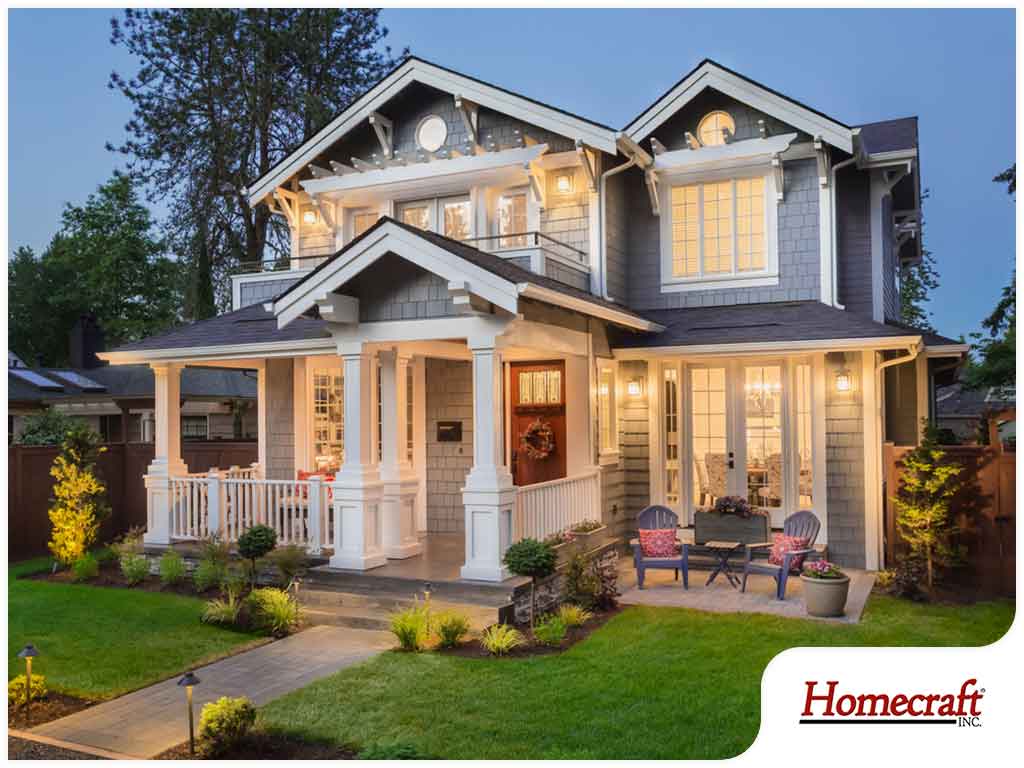This is a photograph of a mid-sized, modern Craftsman-style home situated in a well-populated neighborhood. The house features a perfectly manicured, lush green lawn adorned with neatly arranged flower beds filled with green leafy plants. Leading up to the front porch is a small walkway lined with garden lanterns and shrubs. The front porch, though modest in size and adorned with stout columns, features a white railing and supports a shelter overhead.

The house is distinctively blue-gray with a lot of white trim accenting the windows, doors, and roof. Each window has a thick white border and a small circular window above it, topped with decorative trestles. The two-story structure also includes a balcony on the upper floor, illuminated by two lights. The main entrance features a red door with a wreath, flanked by an old-style mailbox.

To the side of the house, there's another more open patio with two blue plastic chairs and a table between them, each chair decorated with pink pillows. A secondary door leading to the interior is visible behind this seating area, outlined by a white border and illuminated by porch lights.

In the background, there's a glimpse of neighboring properties, including a high brown fence and a large tree, with one neighbor sporting solar panels on their roof. The scene is set against a clear, dark blue evening sky. Notably, in the lower right-hand corner of the image, there is a white section featuring red text reading "Homecraft Inc."